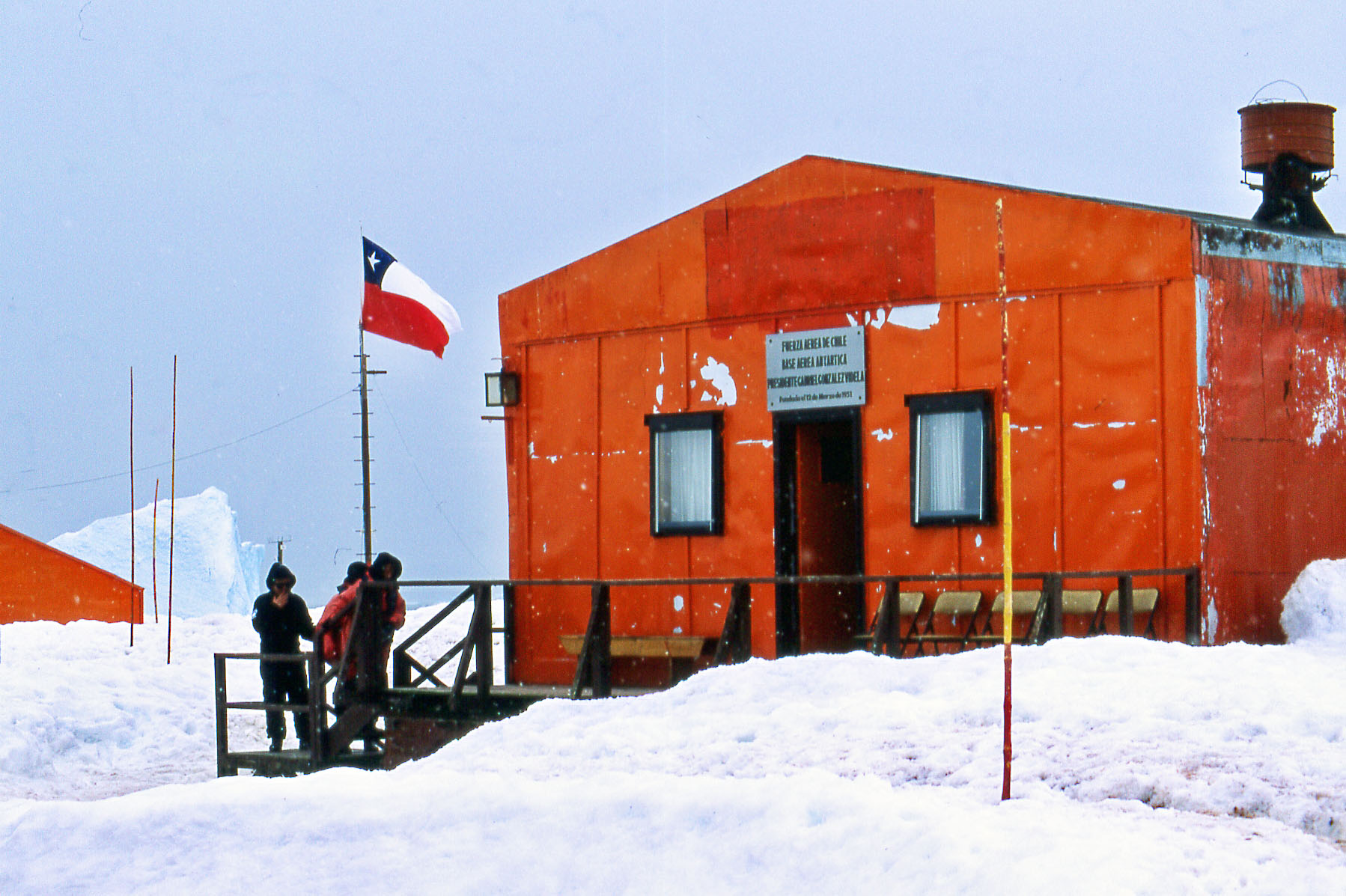The photograph captures a vibrant winter scene at what appears to be a polar research station, characterized by its striking orange, metal-paneled building. The building displays a sign above its entrance, albeit with text too small to read, and features a cylindrical object on its upper right-hand corner. The front facade has two covered windows and an open door flanked by a bunch of folding chairs on a wooden deck. The ground is blanketed in snow, and the clear blue sky enhances the cold setting.

A group of three men, one in a black jacket, another in a red jacket, and a third obscured figure, stand on the stairs leading up to the entrance. They are well-prepared for the winter conditions, each equipped with hoods and goggles. A flagpole stands beside the building, proudly displaying the Chilean flag—distinguished by its white and red stripes and a single white star on a blue square.

In the background, a similar orange building is visible, contributing to the sense of an organized research outpost. This image encapsulates the harsh yet captivating environment of a snowy research station, possibly funded by Chile.